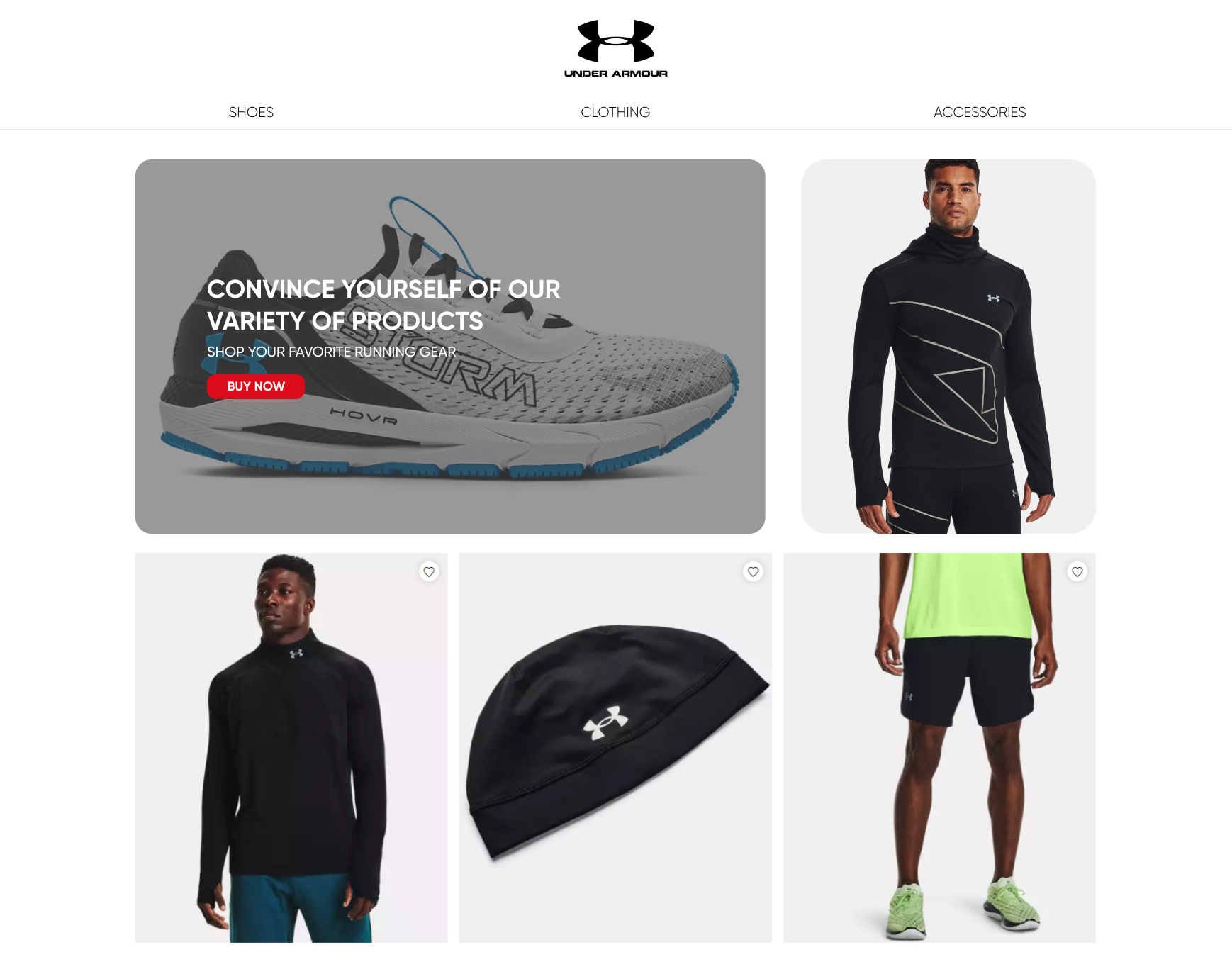This webpage for Under Armour merchandise showcases the brand's logo prominently at the top center, featuring two inverted U's stacked together in black on a white background, with "Under Armour" written below it. Beneath the logo are three navigational tabs in light gray—shoes, clothing, and accessories—each accented by a faint gray line below them.

Below these tabs, the page layout includes one large horizontal rectangle and four smaller vertical rectangles aligned underneath the larger one. The horizontal rectangle, which is the largest, features a dark gray overlay over an image of a shoe named "Nova Storm." The shoe design includes a white front, black heel, white sole, blue rubber bottom, and black laces, indicating it is a low-top tennis shoe. Overlaid in white text is the message: "Convince yourself of our variety of products. Shop your favorite running gear." Below this message is a prominent red button with the white text "Buy Now."

To the right of this horizontal rectangle, the first of the smaller vertical rectangles displays an image of a man with a darker skin tone—possibly Black or Puerto Rican—who is thin, fit, and clean-shaven. He wears a close-fitting, spandex-like black dry-fit outfit with white geometric shapes and the Under Armour logo, appropriate for running.

The second vertical rectangle features a Black man with short, cropped hair. He is dressed in a black long-sleeve dry-fit shirt, which includes the Under Armour logo at the neck, styled like a turtleneck. He also sports blue shorts or pants, which are partially visible.

The third vertical rectangle displays an Under Armour beanie in black with a white logo.

Lastly, the fourth vertical rectangle depicts the lower torso of a Black man wearing a fluorescent green top (visible only from the belly button down), black shorts, and white tennis shoes with either no-show socks or no socks at all. 

This well-structured webpage effectively highlights various Under Armour products in a visually appealing manner, motivating users to explore and purchase items suited for running and athletic activities.